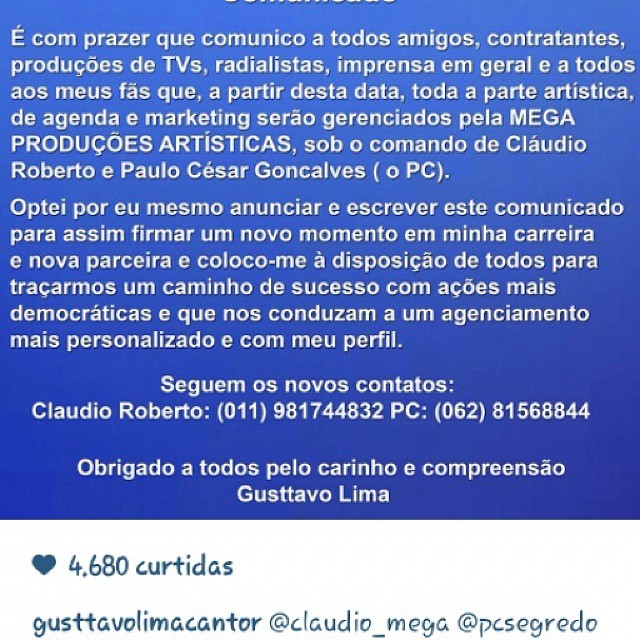The image is divided into two distinct sections. The upper portion, occupying about three-quarters of the space, features a blue background with white text. This text appears to be in Portuguese and reads: "E-C-O-M-P-R-A-Z-E-R-Q-U-E, C-O-M-U-N-I-C-O-A-T-O-D-O-S-A-M-I-G-O-S-C-O-N-T-R-A-T-A-N-T-E-S-P-R-O-D-U-C" among other content. It translates to "It is with pleasure that I communicate to all my friends, contractors." The text includes typical Portuguese grammatical marks absent in Spanish.

The lower fifth of the image also contains blue text, possibly outlining a contact method. It ends with a heartfelt message: "Obrigado a todos pelo carinho e compreensão," meaning "Thanks to all for the affection and understanding," followed by the name Gustavo Lima. There’s more specific contact information present, such as an email address "gustavolimacantor@claudio_mega@p.s.segredo" and a phone number formatted with brackets (011) 98174-4832 and (062) 8156-8844. Additionally, there’s a filled heart icon with the number 4,680 next to it, indicating likes or approval.

In summary, the image is an announcement notice from Gustavo Lima, expressing gratitude and communicating with friends and contractors, and includes detailed contact information at the bottom.